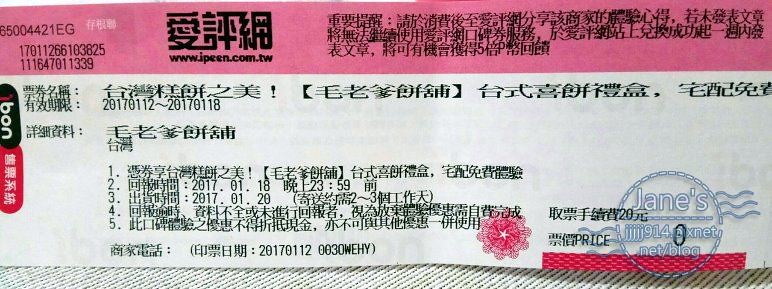The image depicts what appears to be a ticket or a piece of paper with numerous sections, primarily pink, black, red, white, and blue in color. The top portion of the ticket has a distinct pink strip. Adjacent to this pink section on the left-hand side, there are numerous numbers. To the right of these numbers, there is a web address, www.jpeen.com.tw, accompanied by black lettering that is mostly in an Asian language, possibly Chinese or Japanese, making it difficult to decipher.

In the upper left corner, one can discern some serial numbers. Moving towards the bottom right, there is another web address, janesjjj914.pixnet.net/blog, and a watermark which includes the text "Jane's Circle," with waves and the word "Price" incorporated in blue. Below the pink strip, there are two circles; one prominently displays the text "Bon," while the other is filled with Japanese characters. Further down, the document is divided into various sections filled with Asian script, and among these, notable numbers like 2017002-2017008 are present. Specific entries in a list like numbered dates are visible but the detailed contents remain unclear due to the language barrier and the blurriness of the text.